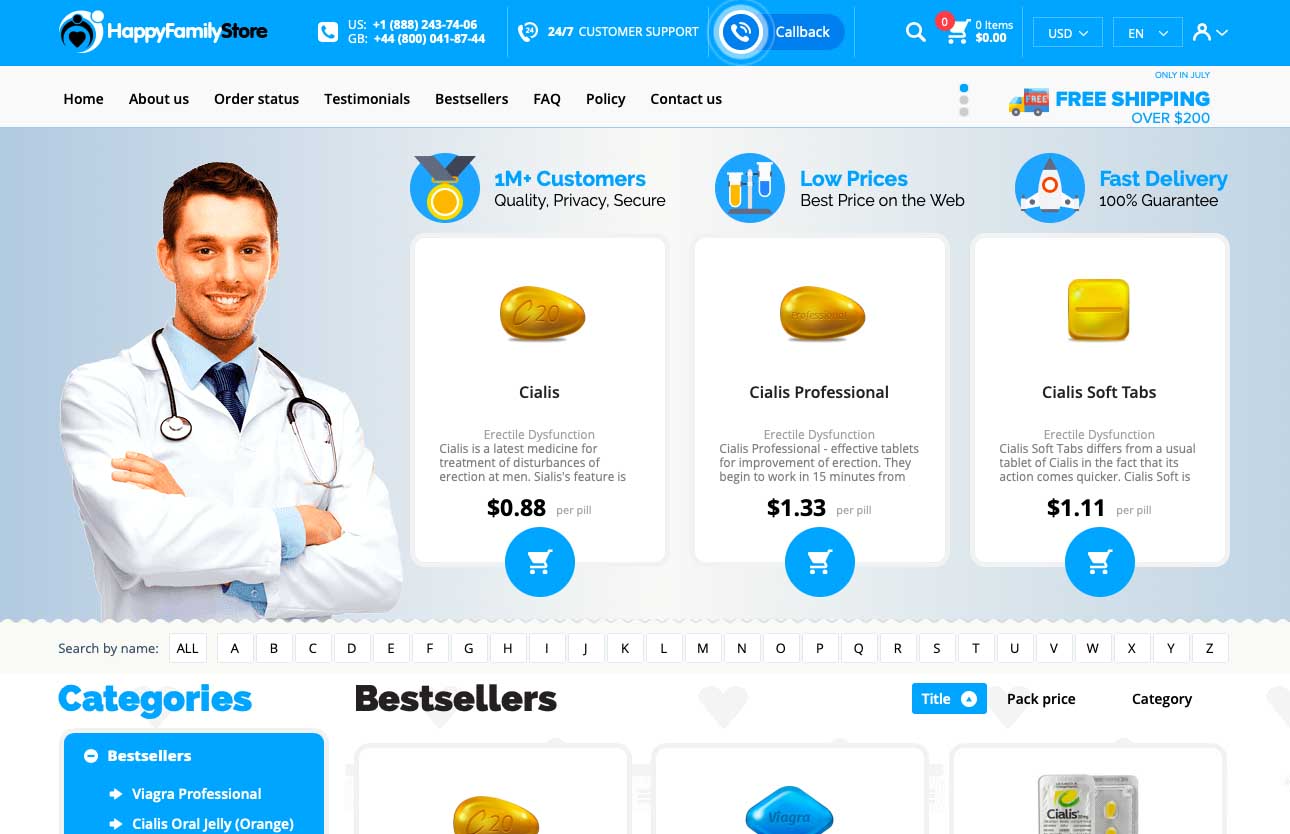This image is a screenshot from a website called "Happy Family Store." The website's emblem is a black heart enshrined within the outline of a person, whose arms extend outward. Surrounding this figure is another person, also outlined, with white dots representing the heads; the arms of these figures curve around like crescents. 

The header displays various navigation options, including "Home," "About Us," "Order Status," "Testimonials," "Bestsellers," "FAQ," "Policy," and "Contact Us." Additionally, it indicates that the user has an empty shopping cart and provides options for language (EN) and currency (USD). There are also US and UK (Great Britain) contact numbers, highlighting availability of 24/7 customer support with an option for callbacks.

The promotional banners boast having over a million customers and emphasize attributes like quality, privacy, security, low prices, and the best price on the web. The products being sold include "Cialis" and "Cialis Professional," with accompanying images of a man in professional medical attire: a shirt, tie, doctor's coat, and stethoscope around his neck.